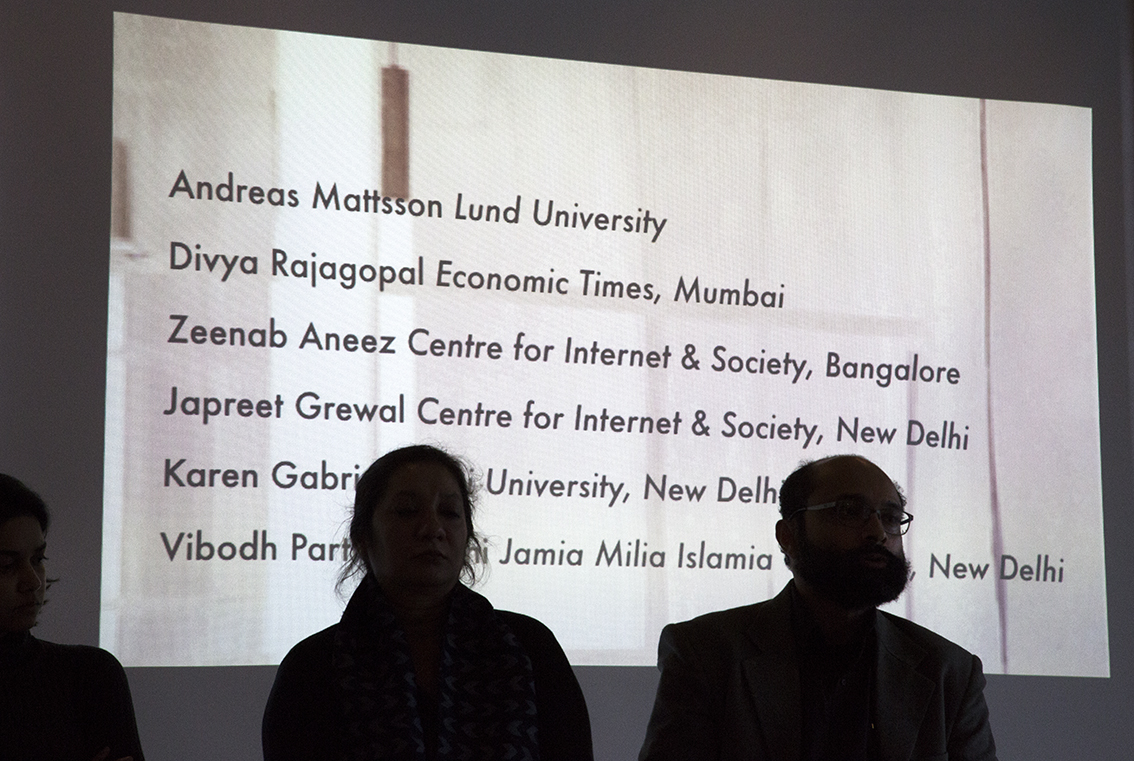The image showcases a projected slide on a white background with black lettering, displaying a list of speakers likely for a seminar or a presentation. At the top, it lists Andreas Mattson from Lund University, followed by Divya Rajagopal from the Economic Times in Mumbai. Next are Zeenab Aniz from the Center for Internet and Society in Bangalore, and Japreet Grewal from the Center for Internet and Society in New Delhi. Two additional names are partially obscured by the heads of audience members: one reads Karan Gabri from a university in New Delhi, and the other starts with Vaibhav Parth from Jamia Mila Islamia in New Delhi. In the foreground, three individuals sit facing the screen, appearing as black silhouettes; the one on the right resembles a male, the middle one a female, and the gender of the leftmost figure is indiscernible.